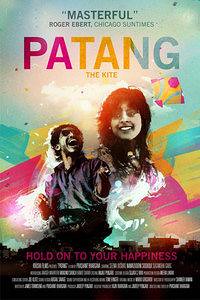This vibrant, colorful movie poster for "Patang (The Kite)" features an out-of-focus mix of pastel watercolors, including magenta, yellow, blue, and orange, creating a cloudy, swatched background. At the top, in various colored fonts, it declares, "Masterful! - Roger Ebert, Chicago Sun-Times." The movie title itself is an artistic blend of cyan, magenta, yellow, and light teal letters. In the center, emerging from the abstract paint strokes, are two figures: a smiling woman with long dark hair, dressed in a white top, positioned slightly to the right, and a man on the left, slightly behind, wearing a blue shirt and glasses with a wide-open grin, possibly holding a kite. Below them, the poster's tagline reads, "Hold on to your happiness," followed by the credits.